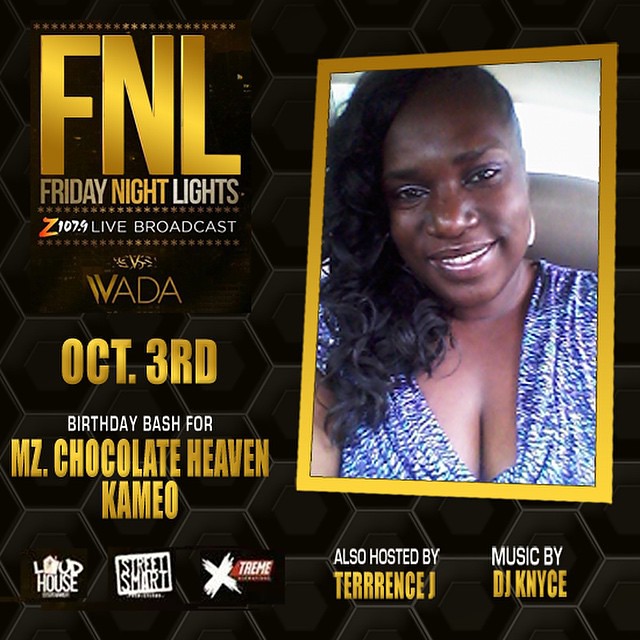The image, a detailed advertisement with a sleek black background adorned with a subtle yellow honeycomb pattern, prominently features a bold gold headline in the upper left corner reading "FNL Friday Night Lights." Below this, it announces a "Z107.9 Live Broadcast." A date, "October 3rd," is listed, marking the occasion as a "Birthday Bash for Ms. Chocolate Heaven Cameo." On the right side, a gold-bordered picture of an African American woman, presumably Ms. Chocolate Heaven, smiles warmly at the camera. She has shoulder-length dark hair and is dressed in a blue outfit, complemented by earrings. Additional details include logos such as WADA, Liquid House, Street Smart Extreme, and text beneath the picture indicating the event is "Also Hosted by Terrence J." with music provided by "DJ Knyce" (spelled K-N-Y-C-E).